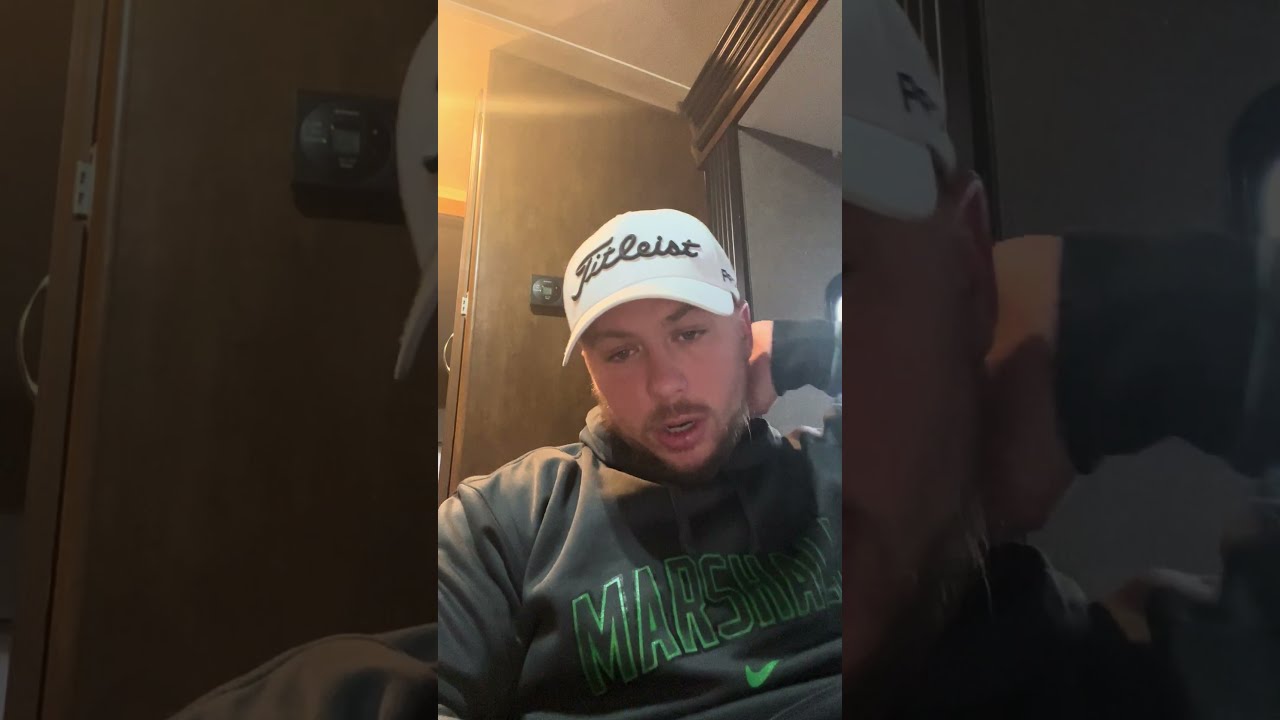The photograph features a teenage male of indiscernible ethnicity, centered in the image. He is wearing a green hoodie with white outlined writing, partially reading "M-A-R-S," though some letters are unclear. On his head is a white baseball cap with black lettering that appears to say "F-I-L-E-I-S-T." The young man has light brown hair mostly hidden by the cap, with visible brown eyebrows, a close mustache, and a very light stubbly beard. His head is tilted downwards and he appears to be looking into a device, either a phone or a laptop, possibly taking a selfie or recording a video, with his mouth slightly open, suggesting he might be talking or smiling. His left hand rests behind his head. The background shows an interior scene with beige walls, what seems to be a white ceiling, and a wood-framed archway or window to the right. Additionally, the image has an overlay, with a zoomed-in and tinted version of his face used as the background, reinforcing the focus on the main centered portrait. He appears relaxed and deeply engaged with whatever is on the device before him.